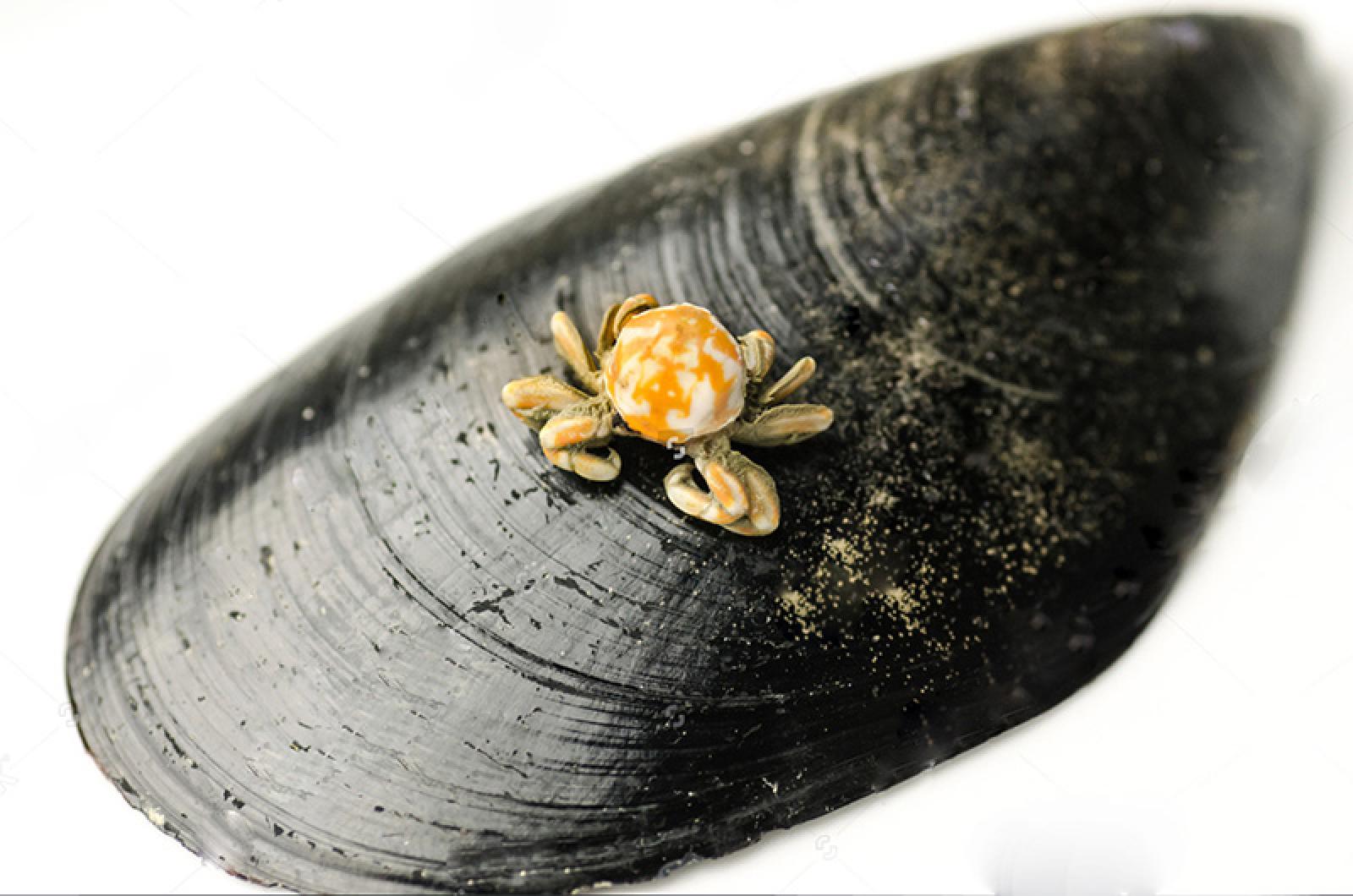This highly detailed up-close photo captures a black oyster shell set against a yellow background, revealing its intricate structure. The shell features definitive lines curving almost horizontally and is adorned with beige specks and streaks, likely bits of sand. Atop the shell sits a tiny crab-like creature, about the size of a thumb, with an orange and white shell. The crab, possibly the inhabitant of the shell, has elongated legs, approximately eight to ten in total, curled up and extending from its body. The shell’s semi-circular lines become larger as they progress towards the left end, highlighting the natural design of the mollusk. The image is zoomed in to prominently display the detailed textures and colors of both the shell and the crab.